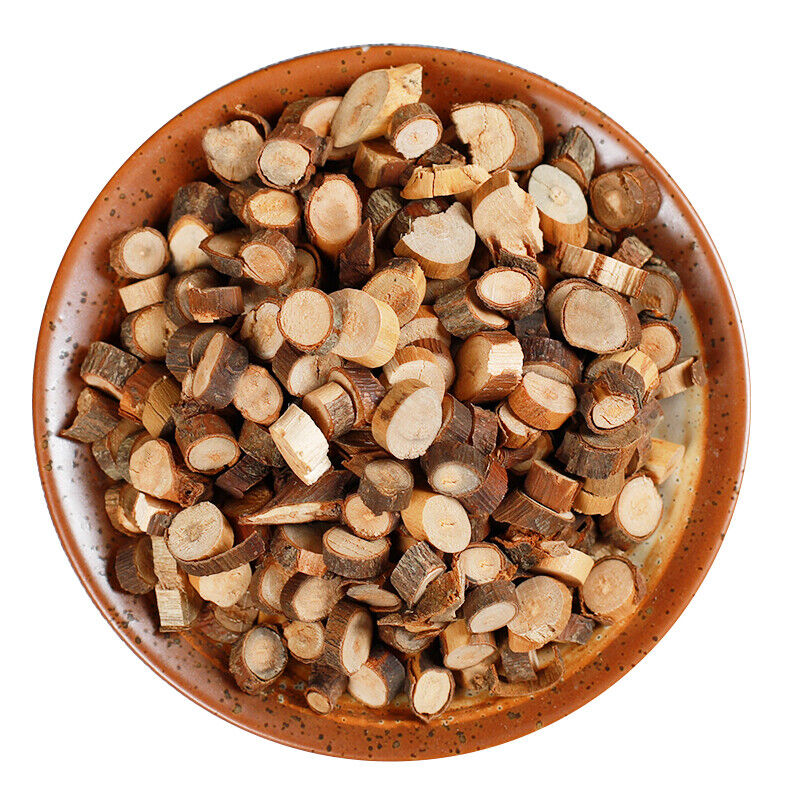The image depicts a close-up, bird's eye view of an orange-ish stone or ceramic bowl with black speckles, resting on a completely white background. The bowl is filled to the top with thin, cylindrical wooden slices of varying colors and sizes, ranging from yellowish to dark brown, and some with orange-ish hues. The wooden slices are intermixed, showing the bark on the edges which contrasts with the lighter sliced surfaces. The slices vary in size, with the smallest resembling coins like dimes and the largest comparable to quarters. The wooden pieces also vary in thickness, averaging about the size of a thick bagel chip. The overall scene suggests a pristine, display-like setup, possibly for sale.